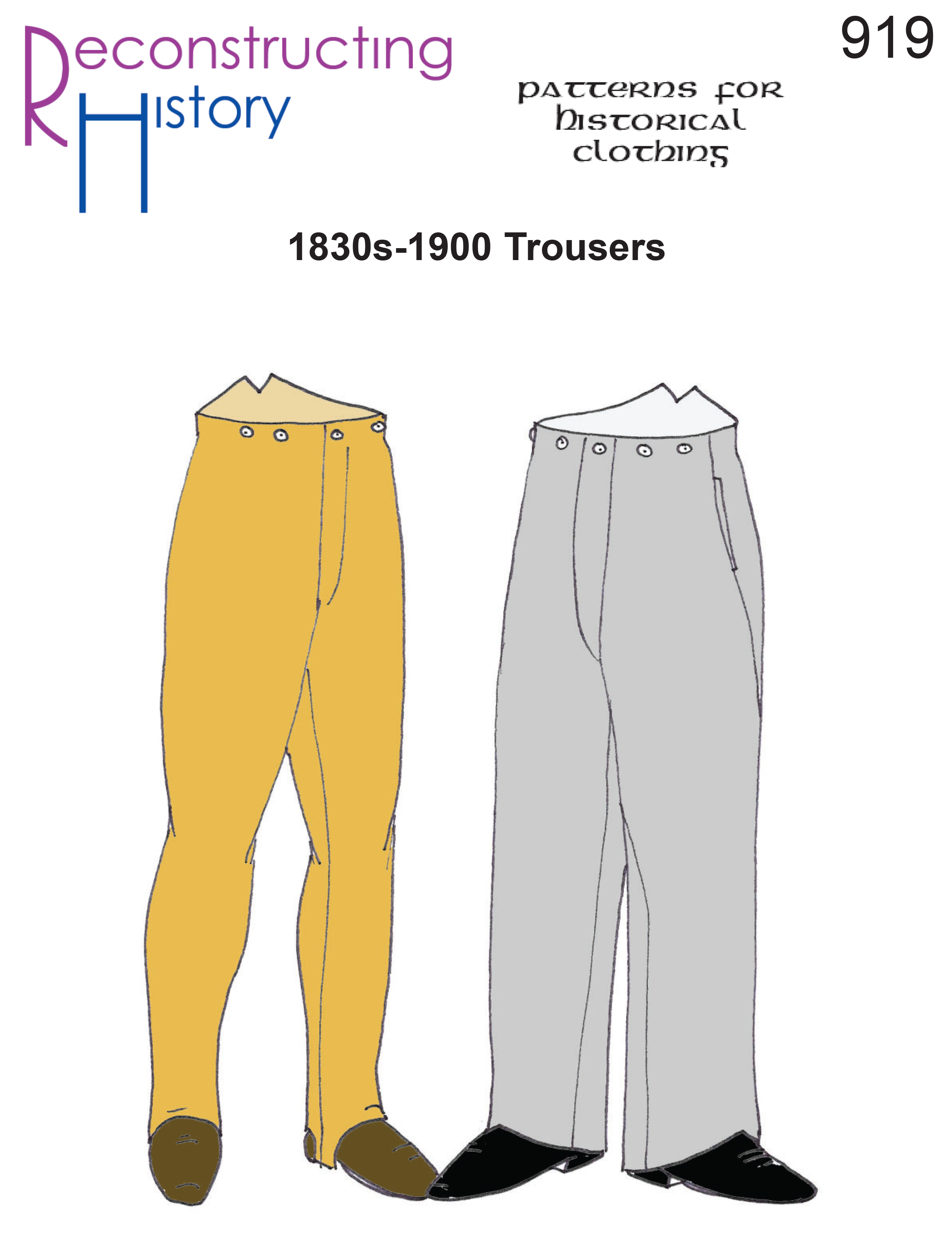This detailed diagram, resembling an advertisement for historical clothing, features two pairs of trousers against a plain white background. The top left corner prominently displays "Reconstructing" in purple text and "History" in blue text below it, with large initial letters. To the right, in a unique font resembling traditional Irish script, it reads "Patterns for Historical Clothing," and the number "919" is positioned at the top right. Beneath this, a bold black text states "1830s-1900 Trousers." On the left side of the image, there is a pair of mustard-colored trousers with four white buttons at the waistband, paired with brown dress shoes. On the right, a pair of gray trousers features five visible white buttons and is accompanied by black pointed dress shoes. Both pairs exhibit a fitted upper section, with the mustard ones being more tapered at the leg and the gray ones providing a looser fit towards the bottom.